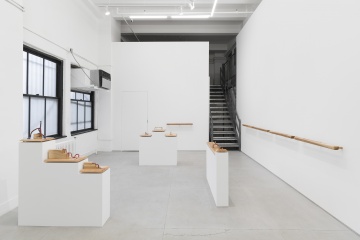This color photograph depicts a spacious and seemingly unfinished gallery or museum installation room characterized by its striking minimalism. The room is dominated by crisp white walls and a clean, smooth cement floor, enhancing the room's bare and open aesthetic. On the left-hand side, two windows with black frames and a pane design allow natural light to filter in. The second window from the front has an air conditioning unit mounted at the top. The right side of the room features a brown wooden banister running along the wall, which leads to a dark-colored staircase ascending into an unseen room, adding a shadowy contrast to the bright setting below.

The room is lit by white fluorescent bulbs lining the ceiling, providing even, diffuse lighting that emphasizes the starkness and cleanliness of the space. Scattered throughout the room are multiple display stands or pedestals made of wood, some tiered with three levels resembling small staircases. These stands hold various undefined objects that might be art pieces or decorative items, contributing to the enigmatic and minimalist feel of the installation. There is no text, no people, and no other furniture, further accentuating the room’s bare and possibly unfinished appearance.